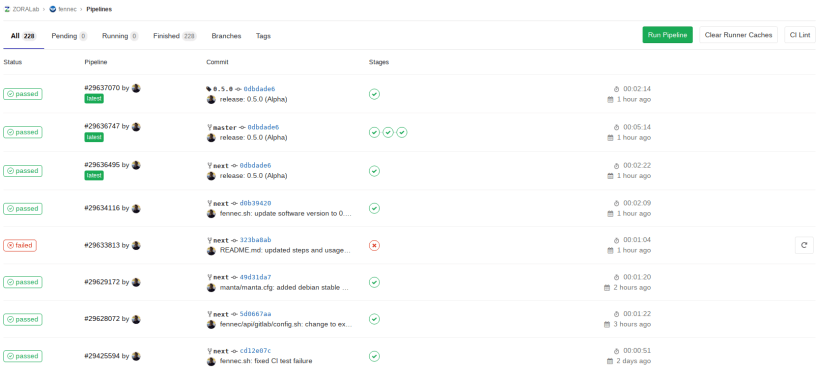The image depicts a dynamic interface of a pipeline management system, characterized by a complex yet organized visual structure. At the top left corner, there is a section featuring grey text on a darker background. Notably, the word "pipelines" is written in black and partially hard to see. Below this header, a grey bar spans across the width of the interface. Under this bar, various statuses are listed in black and lighter text, including "Pending," "Running," "Finished," "Branches," and "Tags."

On the right-hand side, a prominent green button with white text indicates the presence of "1 pipeline." Adjacent to this, two grey buttons display black text, with one reading "Clear Running Cache" (possibly a typo or misheard as "Catch") and the other potentially saying "Lint" or "Weave."

The left section beneath these controls is labeled with headers "Status," "Pipeline," "Commit," "Comment," and "Stages." This area enumerates eight pipeline entries, majority marked with a green "Passed" status. However, the fifth entry stands out in red, labeled "Failed."

The interface further shows specifics of user activity, with entries tied to users identified by numerical IDs like "29637070." Comments and stages are also noted, providing additional context. The right-hand side details the execution duration and timestamps, offering a temporal snapshot of pipeline performance and recent updates.